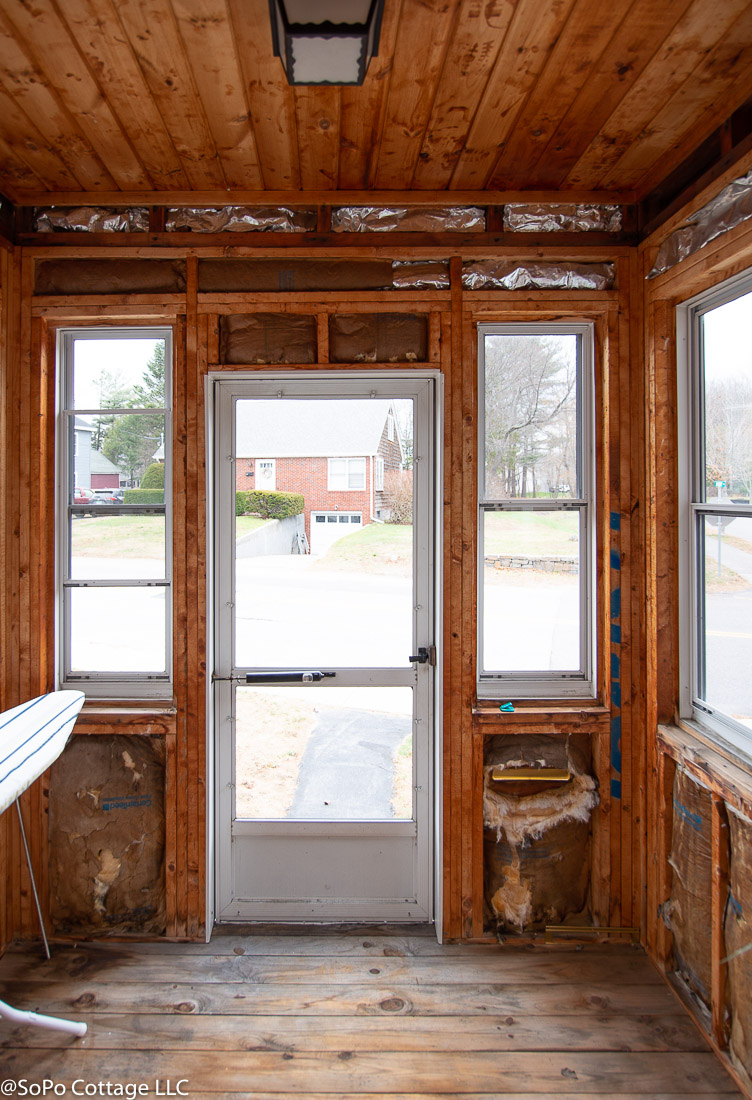This is a vertical color photograph of what appears to be an unfinished or partially renovated back porch in a North American residential area. The image is taken from inside the porch looking out through a screen door, flanked by two tall, narrow windows. The walls are exposed, showing raw wooden beams and torn insulation, indicating incomplete construction. The flooring is made of wood planks, continuing the raw, rustic aesthetic of the space. A wrought iron light fixture with cloudy glass hangs from the pine ceiling, adding to the room’s rugged charm. Notably, there is an ironing board partially visible on the left side of the frame, suggesting the space is still in use despite its unfinished state. Beyond the screen door, one can see snow-covered ground and a neighboring house garage, highlighting the wintry conditions outside. The small room, roughly five to six feet in width, is devoid of much furnishing, save for the visible duct work and the framed-out window on the right wall. The photo was posted by Sopo Cottage LLC.